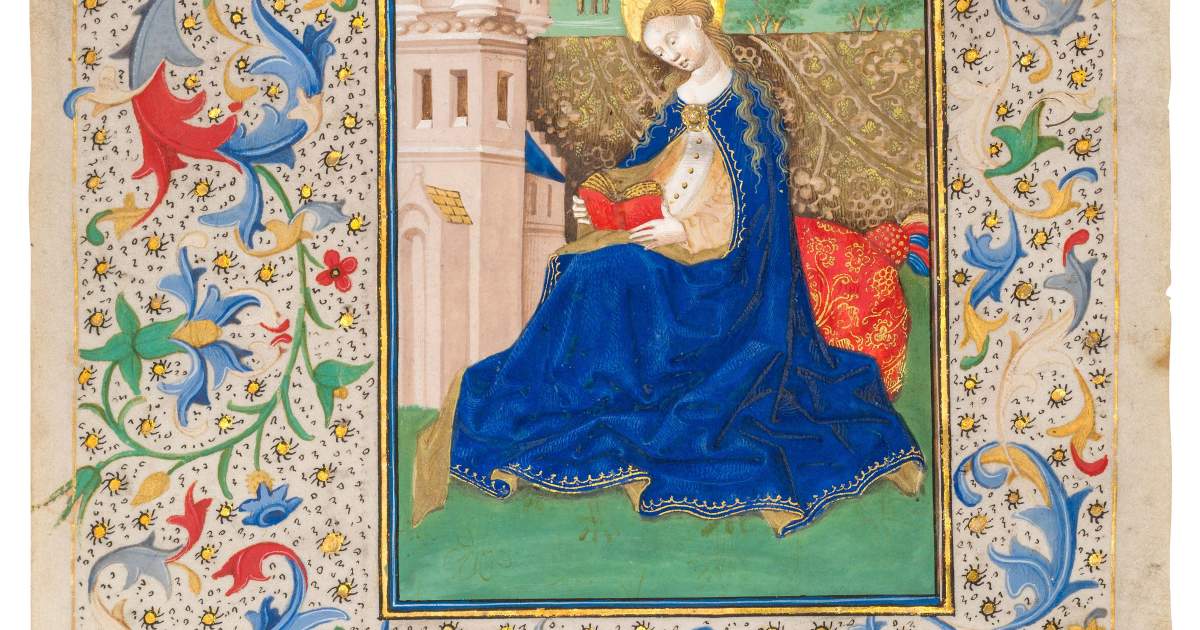This image depicts a medieval-style painting of a saintly woman, centrally positioned. She sits on an intricately embroidered red and gold cushion in a grassy courtyard, possibly outside an ivory-colored building with blue roofs and turrets, indicating a church, abbey, or castle. The woman is adorned in a radiant blue cashmere dress with gold long sleeves and a white placket with buttons, fastened at the neck with a gold brooch. Her long, golden-brown hair, slightly wavy, frames her pale complexion. Her head is bent over a red book with gold pages. Above her head is the lower edge of a halo, symbolizing her saintliness. A light brown patterned blanket hangs behind her. The entire scene is surrounded by an ornate border decorated with stylized flowers in blue, red, green, and yellow hues. The background of the piece appears to be light tan, resembling muslin, and shows slight wear with frayed and stained edges.